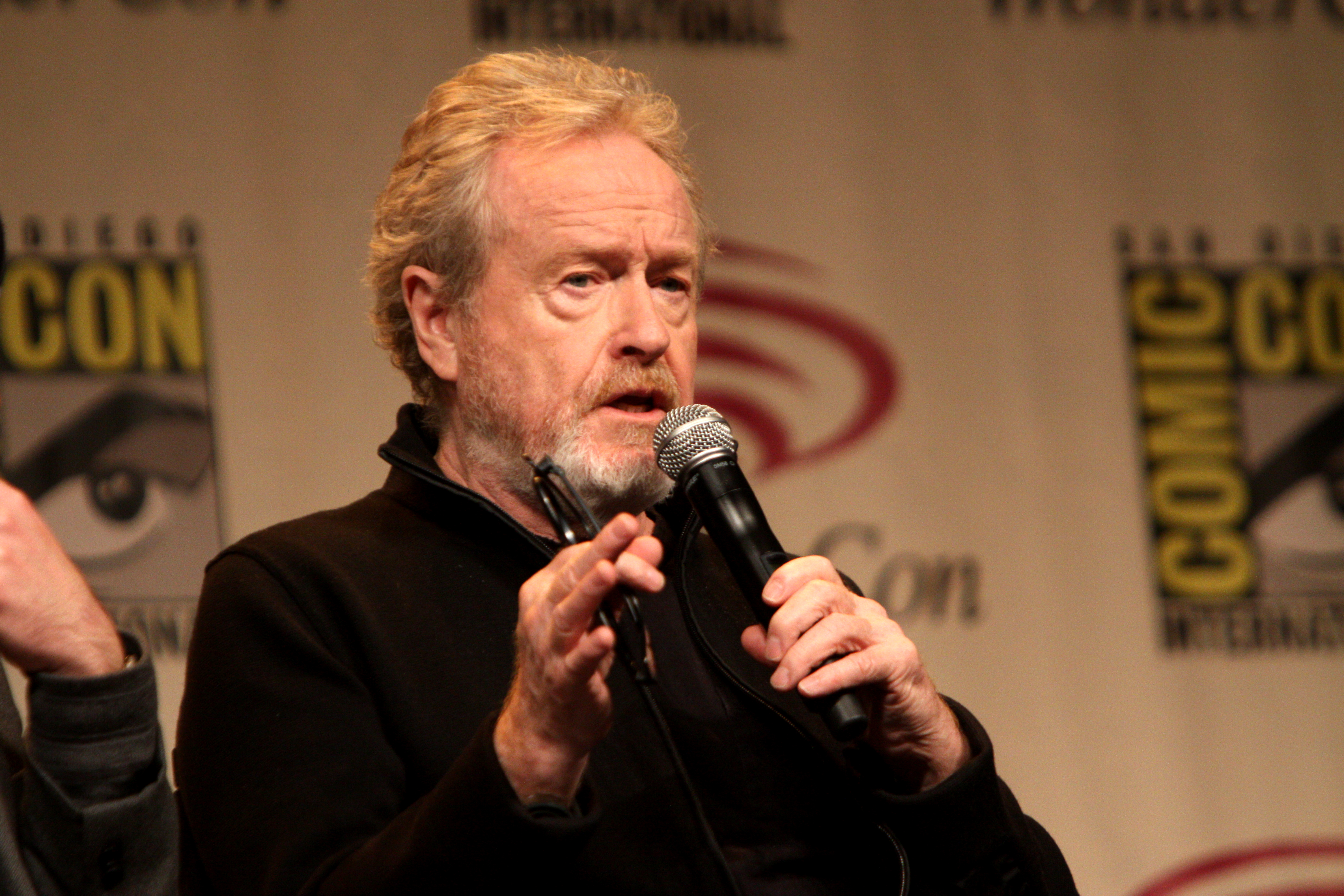In this detailed color photograph, an older man is visible from his chest upwards, speaking into a black microphone with a silver top held in his left hand. He wears a black long-sleeve jacket with a high collar and holds a pair of black-rimmed sunglasses with black lenses in his right hand. The man has a gray beard and mustache, light brown hair—brushed and swept backwards—and noticeable bags under his eyes. He stands before a white wall adorned with multiple Comic-Con logos. To the left, partially out of frame, is the arm of another individual clad in a black leather jacket.